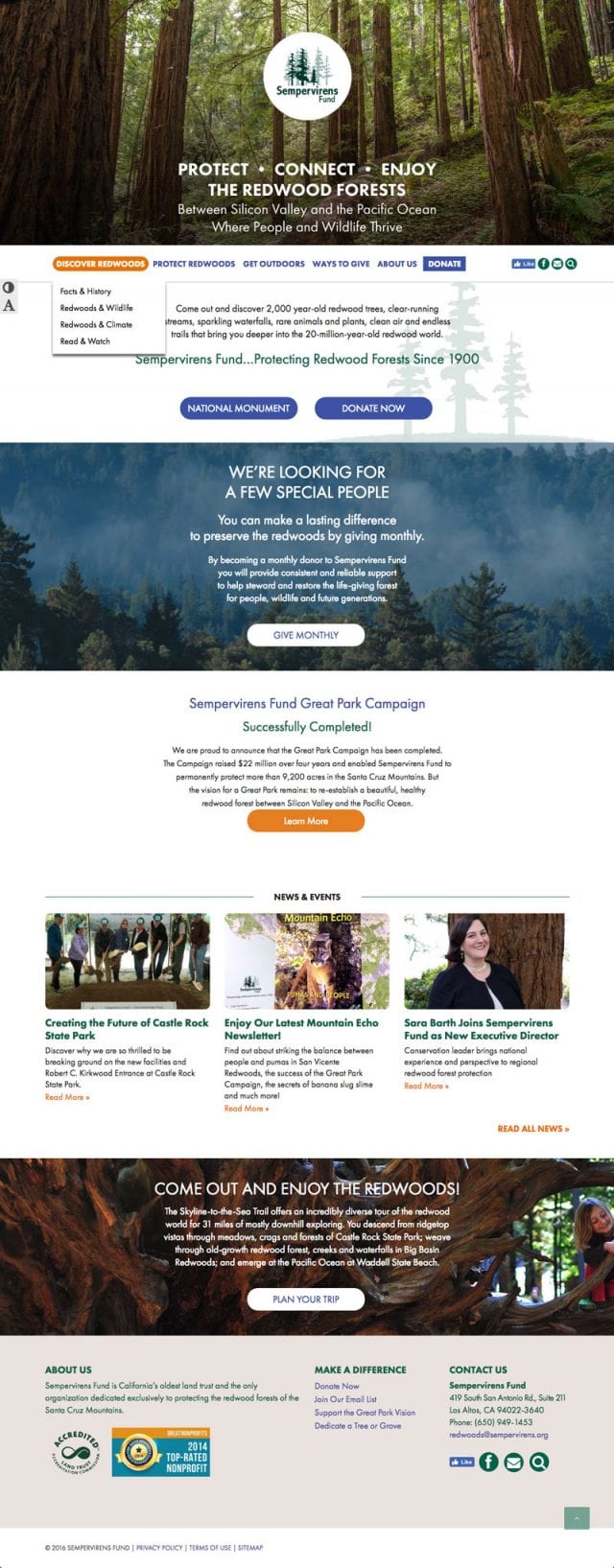**Captivating Image of Sempervirens Fund Website Interface**

This image showcases the homepage of Sempervirens Fund, a conservation organization dedicated to the preservation and enjoyment of redwood forests spanning from Silicon Valley to the Pacific Ocean. The website header prominently displays the organization’s mission: "To protect, connect, enjoy the redwood forest between Silicon Valley and the Pacific Ocean where people and wildlife thrive."

Beneath the header, users are invited to "Discover the Redwoods" through various informative links including facts and history, redwoods and wildlife, red wolves and climate, and multimedia resources for reading and watching.

Further into the website, visitors can find links for more actions such as protecting redwoods, getting outdoors, various ways to donate, and more detailed information about Sempervirens Fund. Engagement options like a Facebook like button, email subscription, and search functionality are readily available.

A highlighted section beckons explorers to experience ancient redwood trees, pristine streams, sparkling waterfalls, and endless trails. It celebrates the Sempervirens Fund's legacy of protecting these marvels since 1900. Users can delve deeper into these treasures through links to the National Monument and donation pages.

The website also features a call to action for monthly donors, emphasizing the significant impact regular contributions can make in preserving these ancient forests. There is a “Give Monthly” button for easy access.

Another section highlights the successful completion of the Great Park Campaign, which raised $22 million over four years and secured over 9,200 acres in the Santa Cruz Mountains. This campaign aims to restore a thriving redwood forest landscape. Users can learn more through an embedded link.

The "News and Events" segment features notable updates, such as the ongoing development of Castle Rock State Park and welcoming Sarah Barth as the new Executive Director of Sempervirens Fund.

Lastly, the website encourages public engagement with the redwoods and offers sections detailing the organization’s history, ways to make a difference, and contact information.